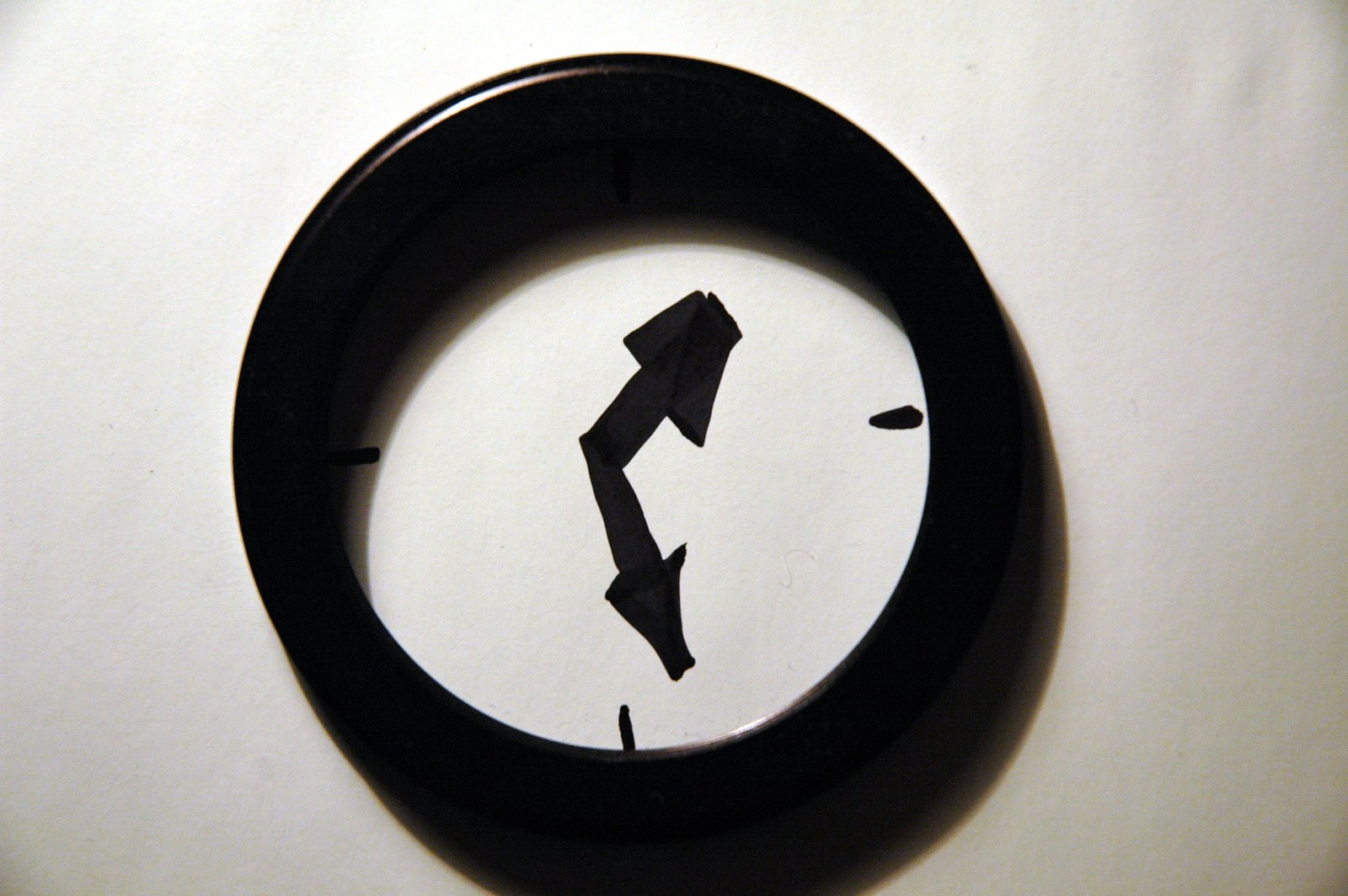The image depicts a circular clock hanging on a smooth white wall. The clock has a boldly defined black border, circumscribing a clean, white face. This face is minimalist, featuring only four small, black spherical marks at the 12, 3, 6, and 9 positions in place of numbers. Thick, black clock hands give the appearance of being hand-drawn, pointing roughly to the 1:30 position. Notably, the clock casts a distinct shadow downward and to the right, enhancing the visual depth. A white highlight on the top left edge of the clock suggests a light source from the top left, adding to the realistic portrayal of shadows on both the wall and the clock's face itself. This striking blend of light and shadow makes it challenging to discern the exact time and gives the impression that the hands and tick marks might be slightly uneven.